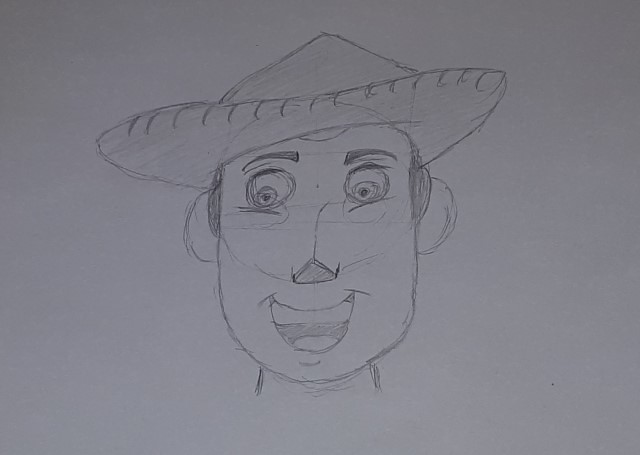This detailed pencil drawing, rendered in black and white on gray paper, captures the head of a man in a rectangular, landscape-oriented frame. The man is depicted wearing a wide-brimmed hat and is shown from the neck up. His expression is joyful, with his mouth open in a broad smile that reveals his top teeth and tongue. His gaze is directed downwards and to the left, adding a sense of dynamism and depth to the portrait.